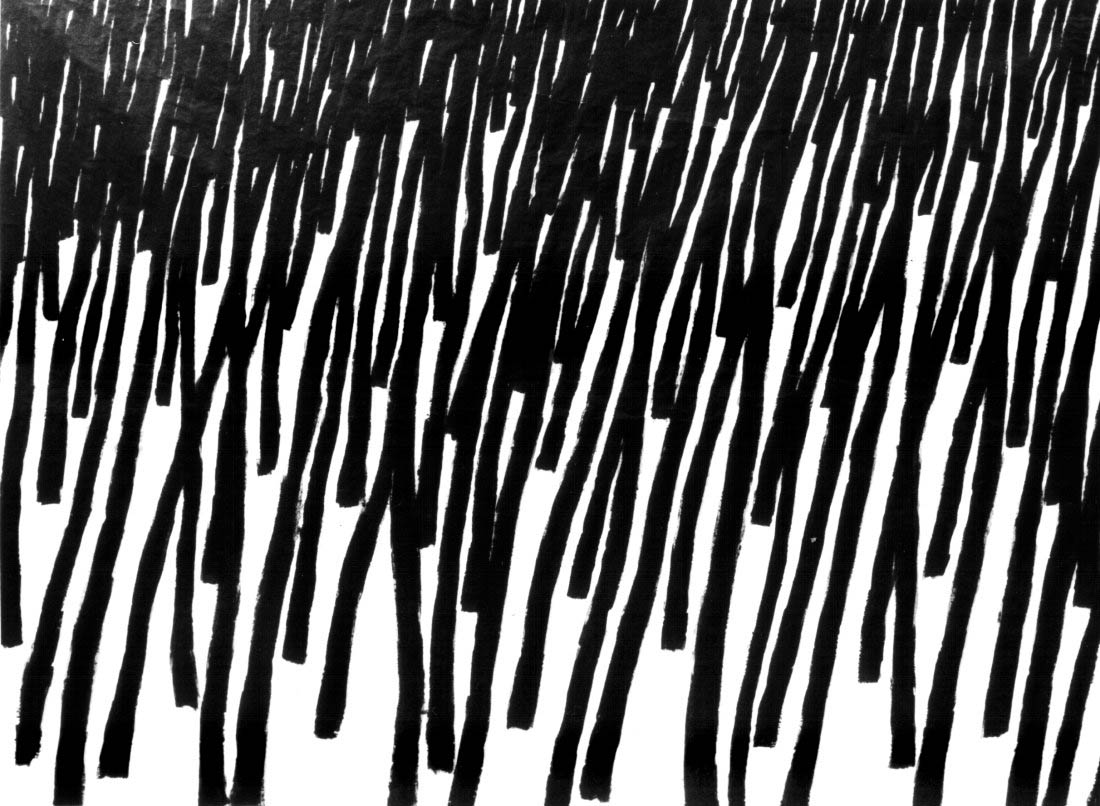The image depicts a dynamic scene characterized by numerous straight black lines emerging from a white base, resembling either hair follicles or vertical black poles. The lines vary in density, being most concentrated in the upper left and upper middle sections, while becoming sparser towards the upper right corner and further decreasing in density from top to bottom. The lines appear to be of differing lengths and are slightly inclined to the right, creating a striped effect against the stark white background. The lines are not uniformly distributed but rather form clusters, giving the image a textured, almost three-dimensional quality. The overall composition captures a striking contrast between the dense, intricate array of black lines and the bare, pristine white background, presenting a visually engaging, monochromatic pattern.